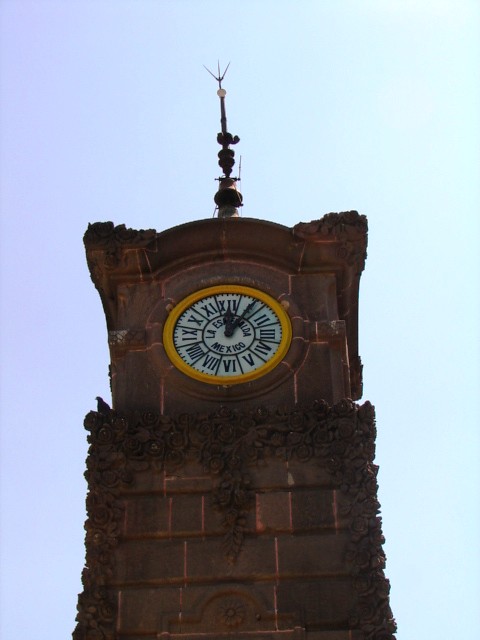The image captures an outdoor scene featuring a majestic clock tower set against a clear, light blue sky, emphasizing the upward perspective. The clock tower, constructed from large, dark brown-reddish bricks with white mortar lines, showcases a sturdy and historic appearance. The lower section of the tower is slightly wider than the upper section, adding a robust base to the structure. Notably, the entire border of the tower is adorned with ornate brown rose-like carvings, enhancing its intricate architectural details.

In the middle section of the tower, there is a slight overhang, while the upper section tapers into an archway. The clock face itself is prominently round, bordered by a yellow circle and featuring a white background. The clock displays time with black Roman numerals from 1 to 12 and black hands, currently reading approximately 12:08. The clock face includes some text, with "Mexico" clearly visible at the bottom, though the text at the top is not discernible. At the pinnacle of the tower, an antenna extends upward, completing the stately and historic look of this clock tower.